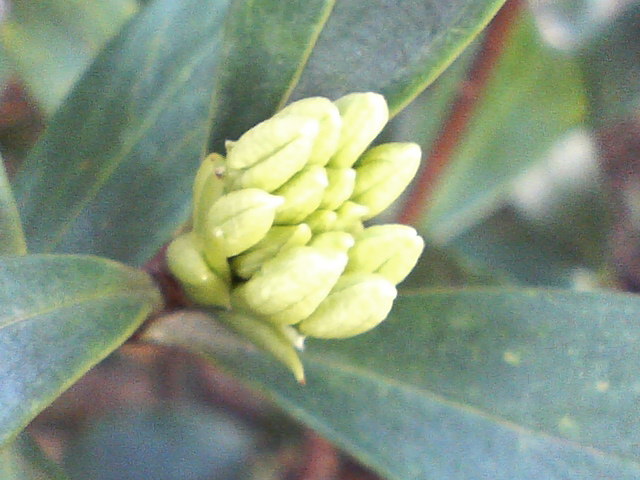This detailed close-up photograph captures a plant that's on the verge of blooming. At the center of the image, a cluster of 10 to 15 cream-colored buds is tightly packed together, nestled in the heart of the plant. These buds are yet to develop into flowers, creating a sense of anticipation and potential growth. Surrounding these buds are three large, pale green leaves that add to the plant's lush and vibrant appearance. The background of the image is intentionally blurred, highlighting the intricate details of the buds and leaves in the foreground. Despite the blur, the background still reveals the presence of additional plant structures, emphasizing the natural setting. This focused composition brings attention to the imminent blossoming of the plant, capturing a moment of natural beauty and growth.